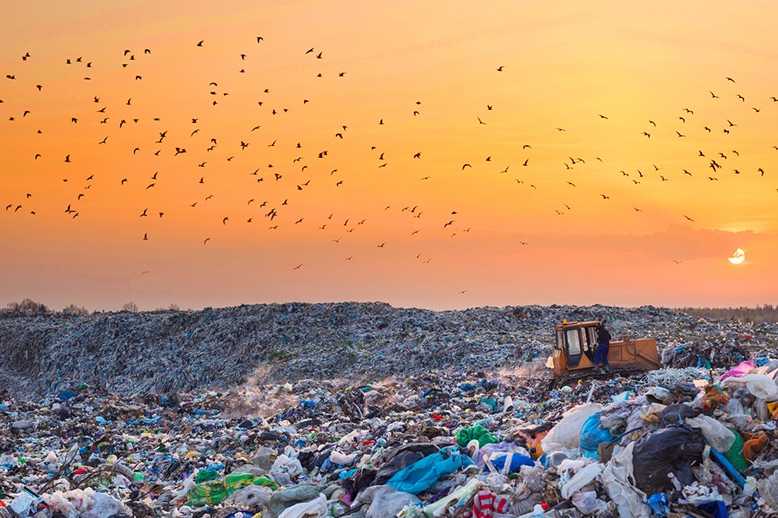The photograph captures a sprawling garbage dump that covers the entire bottom two-thirds of the image. The dump, filled with a chaotic mixture of plastic bags, clothes, and various debris in different shades of blues and reds, stretches out like an endless field of trash. In the center of this chaotic scene, an orange or yellow bulldozer, possibly spreading or compacting the garbage, adds to the industrial feel. Rising from the garbage-strewn landscape is a small hill that forms the horizon. Above this grim spectacle, a stunning sky painted in three tones of orange and yellow illuminates the scene, indicating that the day is about to end. The sunset casts a golden glow, with the sun appearing as a small dot near the horizon. Hundreds of birds are in flight, their dark shapes contrasting sharply against the vibrant sky, adding a dramatic touch to the otherwise somber image.